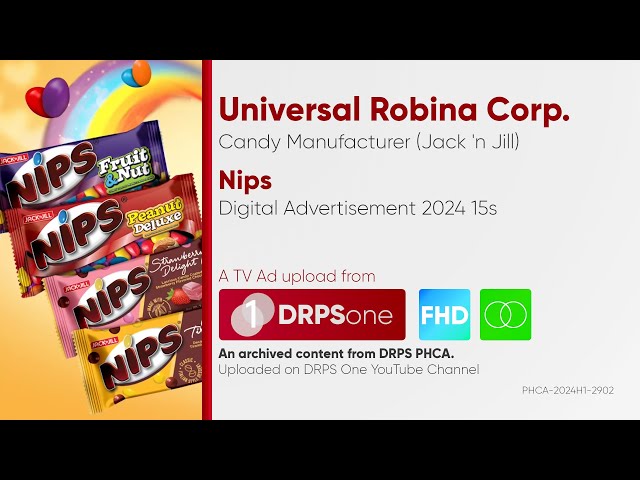This image is a computer-generated digital advertisement for Nips candy by Universal Robina Corporation. The vibrant design features a yellow background with a prominent rainbow on the top left corner. Floating around the rainbow are individual pieces of Nips candy, highlighting four different packages arranged vertically on the left side: Nips Fruit and Nut, Nips Peanut Deluxe, Nips Strawberry Delight, and a partially obscured yellow package whose flavor cannot be identified. 

On the right side, detailed information about the advertisement is provided: "Universal Robina Corp." appears in red, followed by "Candy Manufacturer (Jack and Jill)" in black. The word "Nips" is boldly printed in red beneath. Continuing, it states "Digital Advertisement 2024-15S" in black text, followed by a description of the ad's upload status: "A TV ad upload from DRPS1 FHD." The notation "an archived content from DRPSPHCA uploaded on DRPS1 YouTube channel" is also included to emphasize the digital archival. In the lower right-hand corner, another reference "PHCA-2024-H1-2902" is visible, connecting to the date and other identifiers.